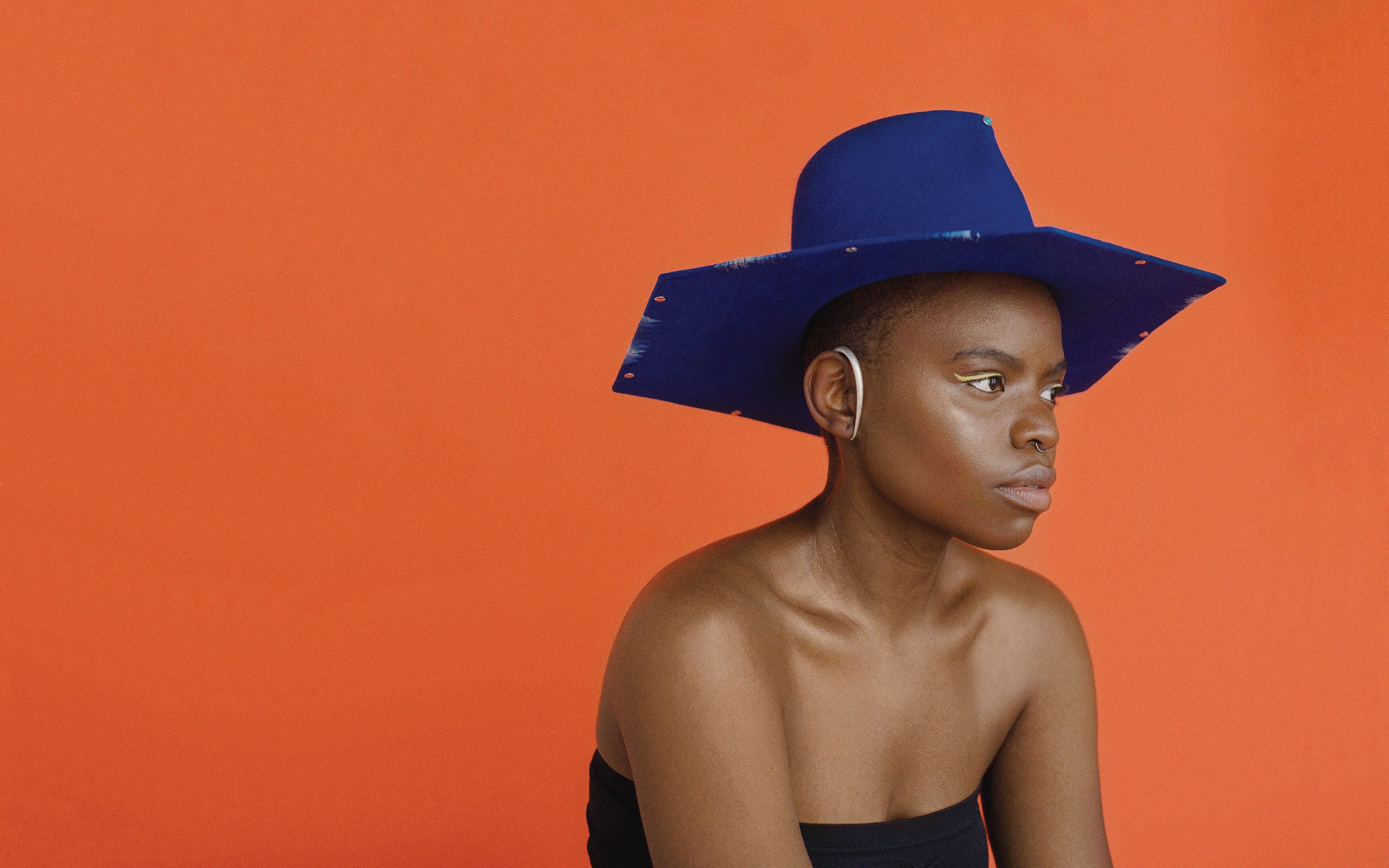The image depicts a dark-skinned African-American girl, seated and shown from the chest up against a vivid orange background. She’s slouching slightly and gazing pensively to the side. She has a shaved head on the sides, with the top covered by an indigo-colored hat featuring large, irregular geometric shapes. Her shoulders are bare, leading to a tube-like black top or dress that leaves her upper chest exposed. A notable feature is a white device or band, potentially a listening device, latching around her ear from front to back. She sports a striking nose ring that connects both nostrils, and there's a subtle hint of dark eyeshadow on her eyelids. Her features include a broad nose, thick eyebrows, and full lips, and the image captures her model-like poise, emphasizing the muscles of her shoulders and neck.